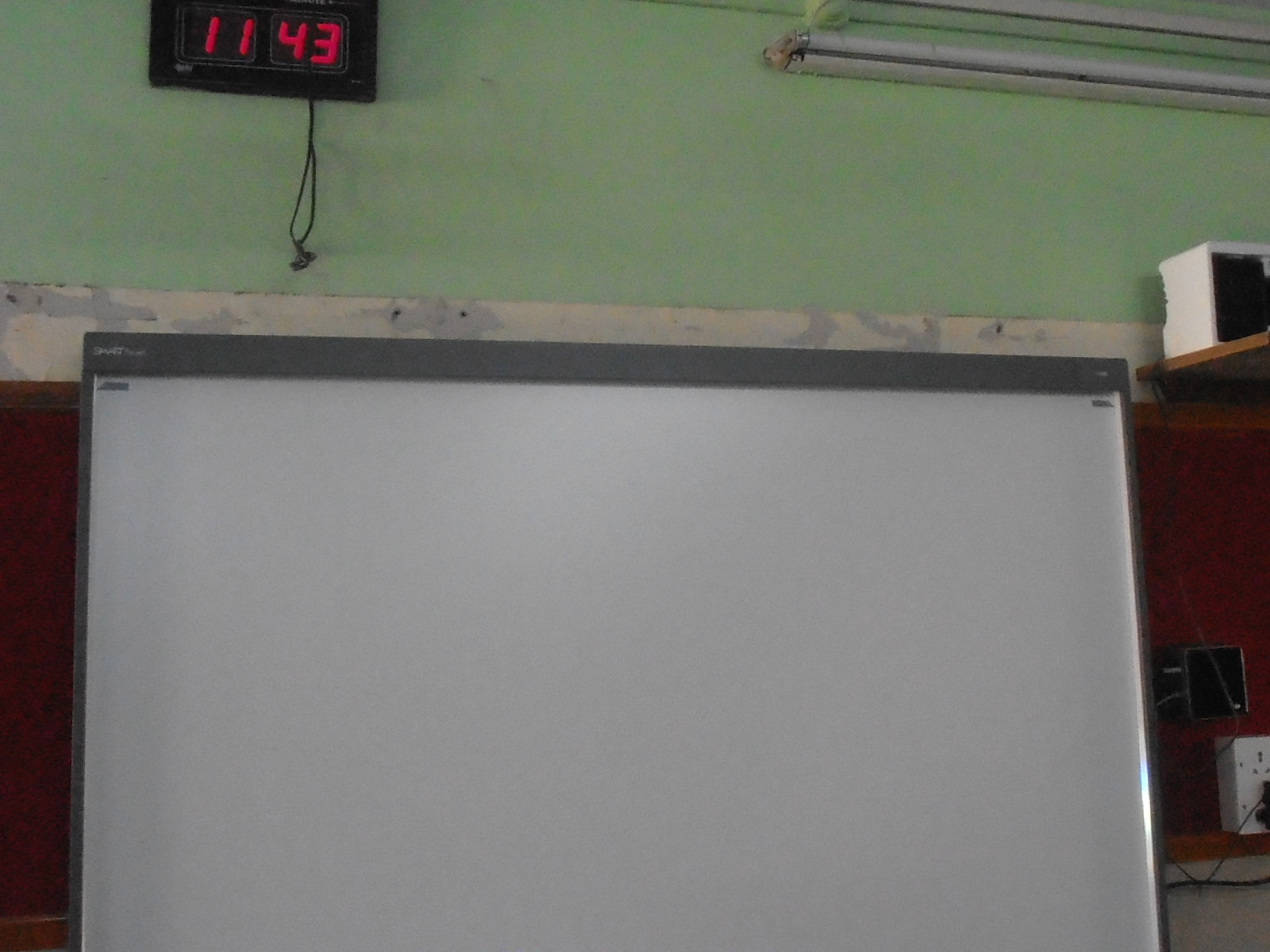The photo captures the interior of what appears to be a classroom with very dim lighting, viewed from a slightly upward angle focusing on a section of the wall. Dominating the scene is a smart board, characterized by its dark gray thin frame surrounding a white center, though it is not turned on. Above the board, the wall is painted a mint green color. In the upper left portion of the image, a rectangular black digital clock displays the time as 11:43 in red numbers. The bottom part of the smart board is cut off, showing only about three-quarters of it. To the right, the wall features some brown wood paneling around a section that might house an unused LED x-ray viewing box or bulletin board. Adjacent to this, there are shelves with various items, including a black and white object that resembles a fan or some technological devices, perhaps modems or routers. The image captures the typical technological setup of an educational environment.